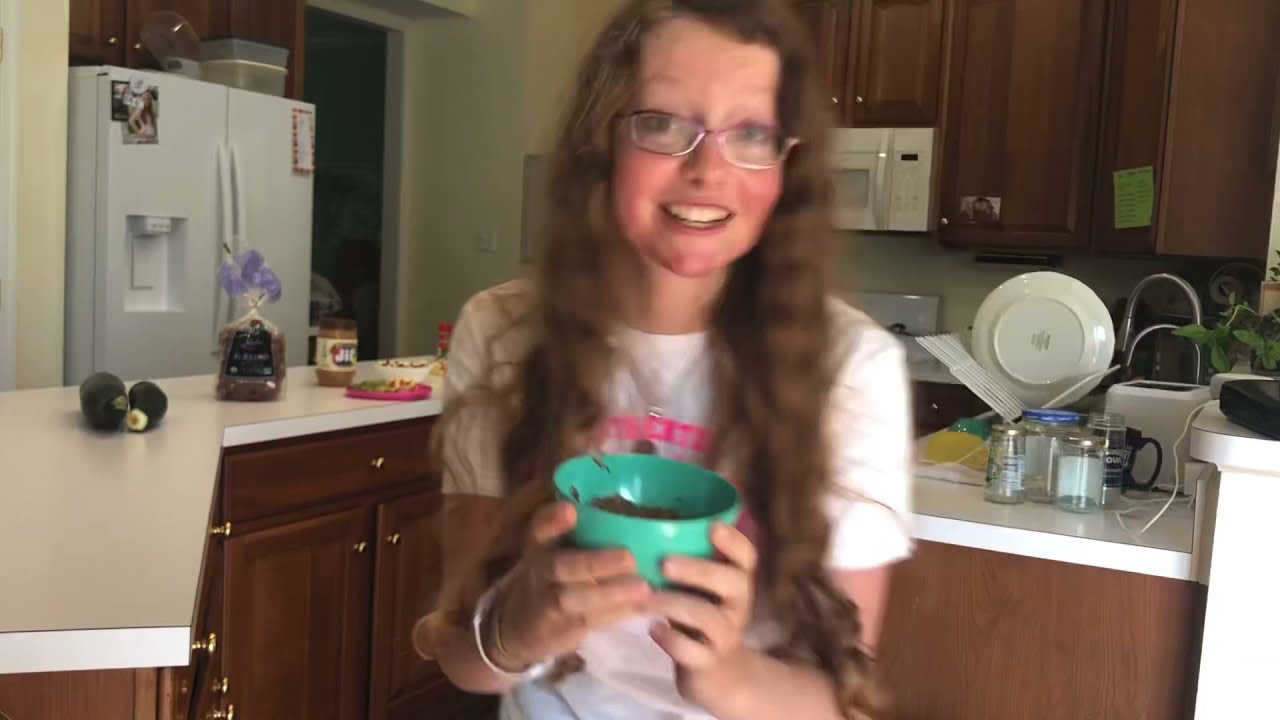In the center of a brightly lit kitchen, a woman with long, wavy brown hair cascading past her elbows stands holding a turquoise bowl filled with a brown substance. She is smiling and wearing glasses with purple rims, a white shirt with pink, unreadable lettering, and a silver necklace and bracelet. The kitchen behind her features a mix of white and wooden elements. To her left, a white refrigerator adorned with a photograph of a football player stands next to an L-shaped island with a white countertop, on which dark green vegetables, a bag of bread, a jar of Jiffy peanut butter, and a purple plate are visible. Below the island are black cabinets. On the right, overhead wooden cabinets house a white microwave, beneath which a light green stick-it note is stuck. Under it, dishes, including a white plate and some clear glasses with silver caps, are drying in a white dish rack next to a white toaster. The countertops around her are white, and the kitchen walls are a light beige with a slight yellow tint.